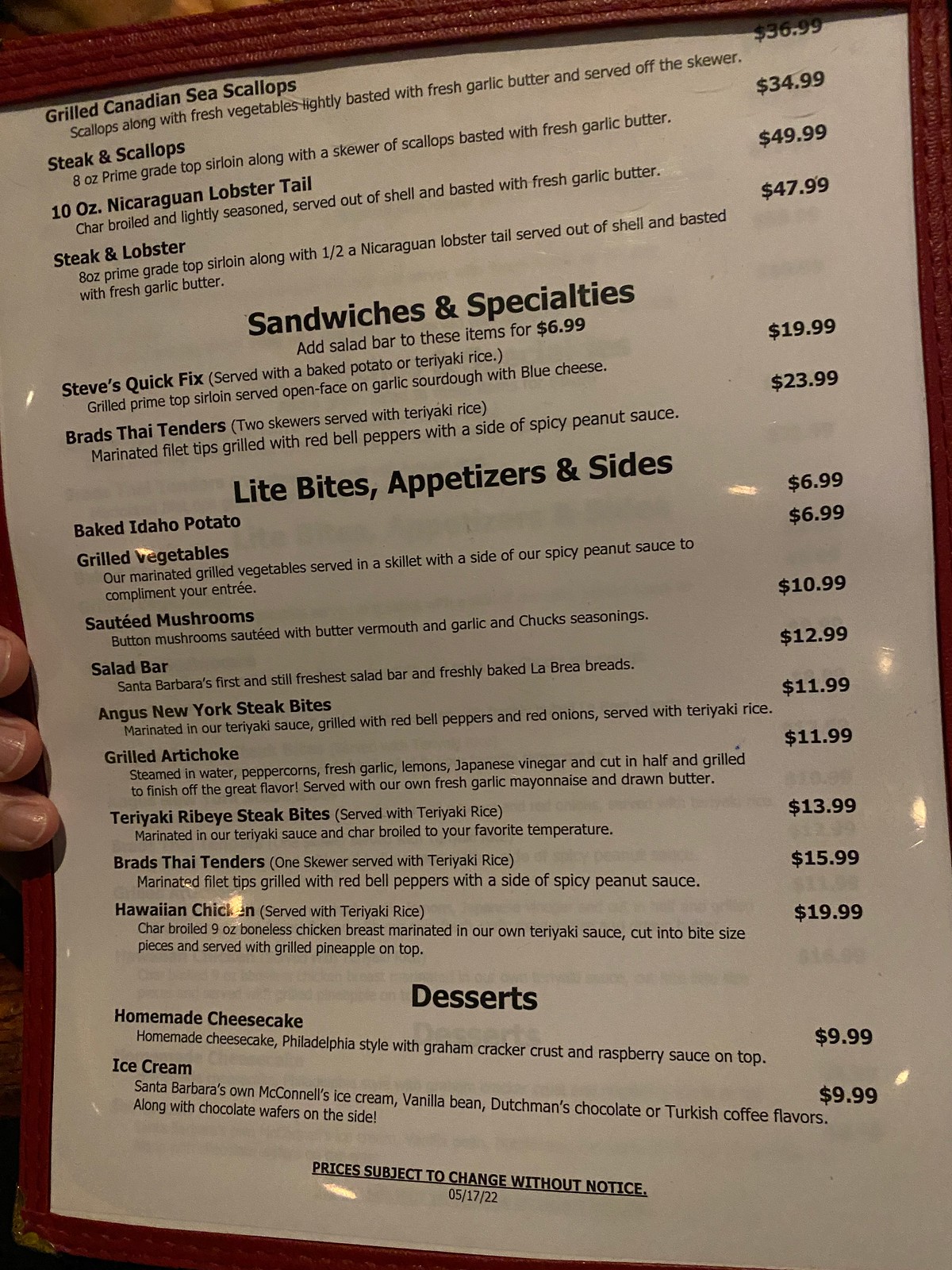Indoor color photograph of a menu with approximately 20-23 items. The top of the menu is not visible, leaving the establishment unidentified. The visible menu is organized into various sections. The first subheading, "Sandwiches and Specialties," is written in black lettering, under which two items are listed. Below this, the subheading "Light Bites, Appetizers, and Sides" lists several options. Near the bottom, the section labeled "Desserts" is visible.

The menu follows a classic format with food descriptions on the left and prices listed in U.S. dollars on the right. The menu is being held down by three fingertips visible on the left edge.

Items listed on the menu include:

**Top Section Items:**
- Grilled Canadian Sea Scallop
- Steak and Scallops (10 oz.)
- Nicaraguan Lobster Tail
- Steak and Lobster

**Sandwiches and Specialties:**
- Steve's Quick Fix
- Brad's Thai Tenders

**Light Bites, Appetizers, and Sides:**
- Baked Idaho Potato
- Grilled Vegetables
- Sautéed Mushrooms
- Salad Bar
- Angus New York Strip Bites
- Grilled Artichoke
- Teriyaki Ribeye Steak Bites
- Brad's Thai Tenders
- Hawaiian Chicken

**Desserts:**
- Homemade Cheesecake
- Ice Cream

Each item is followed by its respective price in the right-hand column.